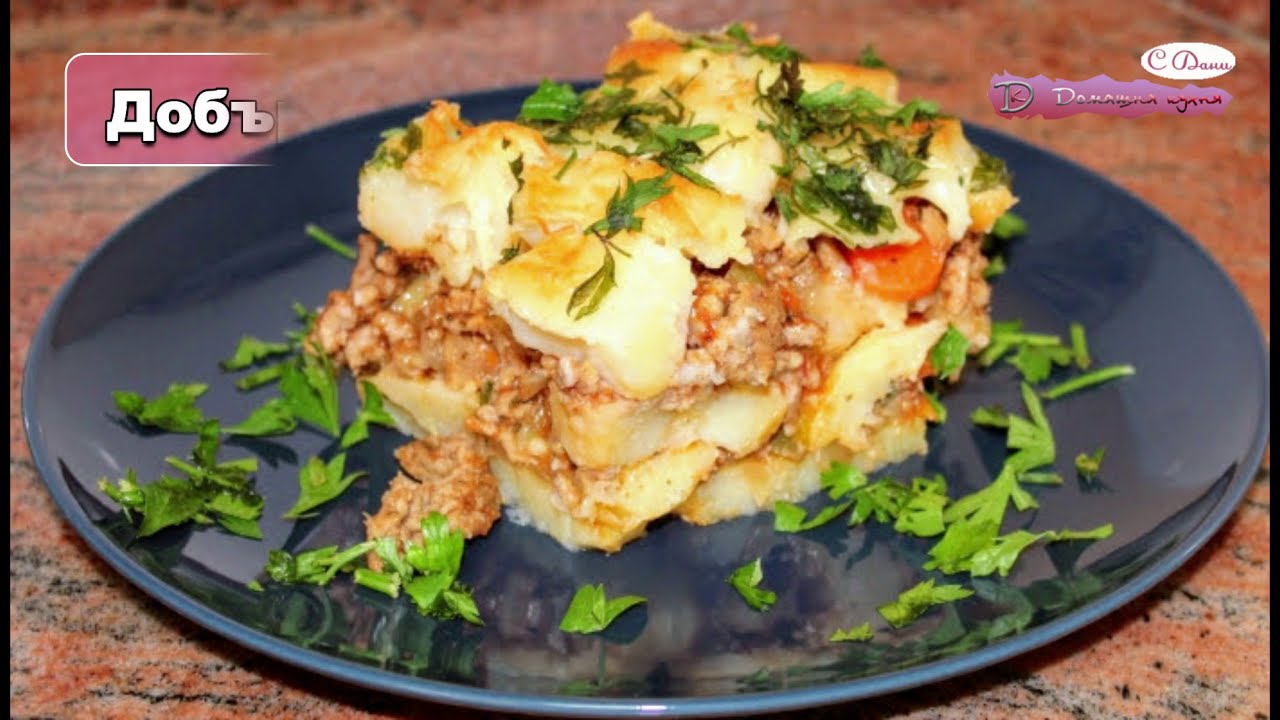This image depicts a close-up view of a tantalizing, layered dish presented on a glossy black plate, placed atop a reddish-gray-black granite table that reflects light off its polished surface. The central portion of the dish features a hearty combination of crushed individual biscuits or rolls forming a base, topped with a substantial amount of ground beef, which varies in size from large chunks to smaller pieces. Atop this robust layer, bits of what appears to be tomato are visible, complementing the savory meat. The entire creation is garnished with scattered pieces of fresh lettuce and possibly parsley, adding a vibrant green element to the visual appeal. Fine black spices are sprinkled across the dish for an added touch of flavor and aesthetics. Encircling this culinary ensemble is an overlay of text, indicating some sort of labeling or identifier, with "A06B" inscribed in white within a fuchsia background on the left side, and "C. Davis" in black text inside a white oval, alongside some partially obscured text on the right. This plate of food suggests influences from Middle Eastern or Italian cuisines, potentially presented as part of a web-based cooking show or food review, as inferred from the structured text labels.